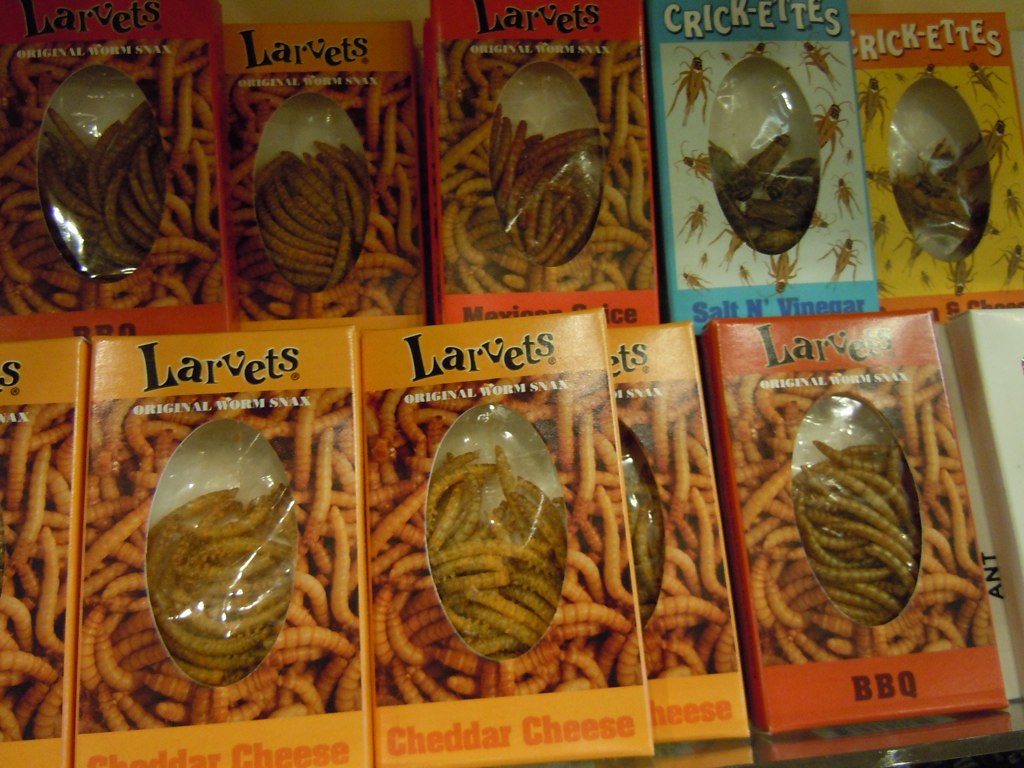The photograph showcases a display shelf filled with a variety of packaged edible insect snacks. On the lower shelf, the main focus is on "Larvets," the original worm snacks, which come in bright yellow to red packaging featuring a clear plastic cutout that reveals the fried mealworms inside. Notable flavors include cheddar cheese on the left and barbecue on the right, with the worms appearing more distinct in the barbecue packaging. Additionally, you can see "Crickettes" in blue boxes prominently labeled with flavors like salt and vinegar, as well as a less clear flavor that might include cheese. Each box is roughly the size of a deck of cards and has a transparent oval window that displays the contents—either mealworms or crickets, each illustrated on the box for clarity. The products are neatly arranged on what appears to be a white table, showcasing their diverse variety in flavors and insect type.